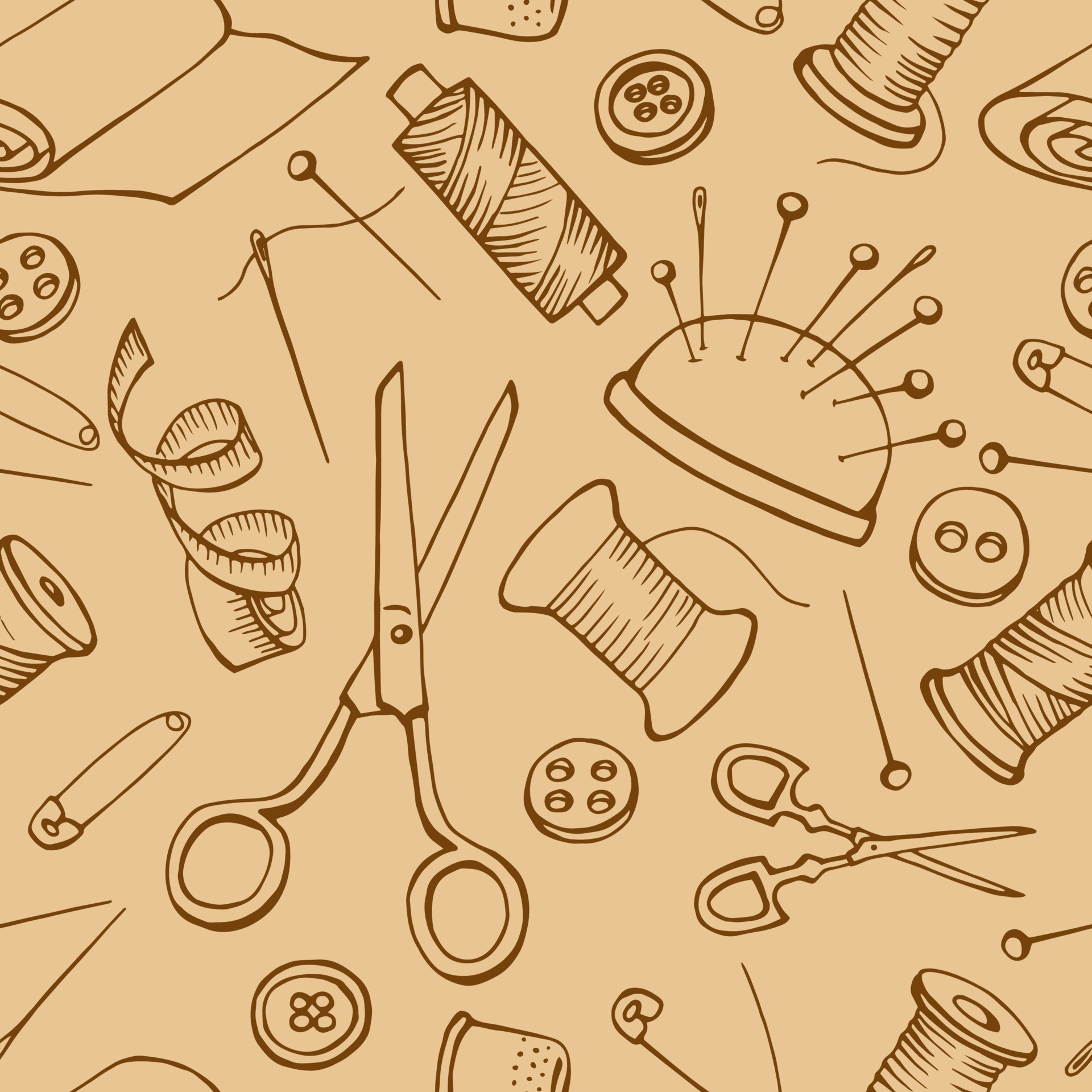This artwork depicts an intricate arrangement of needlework tools, rendered in two tones: a very light brown for the background and a darker olive brown for the detailed outlines. Featuring an array of sewing essentials, the illustration includes various needlework tools spaced throughout the image. Prominently positioned items include a large pair of scissors alongside a smaller one, several needles and pins, a pin cushion bristling with needles and pins, and numerous buttons, some with two holes and others with four. The artwork also showcases a few spools of thread, a measuring tape, and safety pins. There's even a thimble, detailed twice, as well as fabric rolls. The objects are scattered evenly across the image in a somewhat whimsical, cartoonish style, giving the impression of a wallpaper design. Each item is carefully drawn, emphasizing the essence of needlework in this skillful and detailed composition.